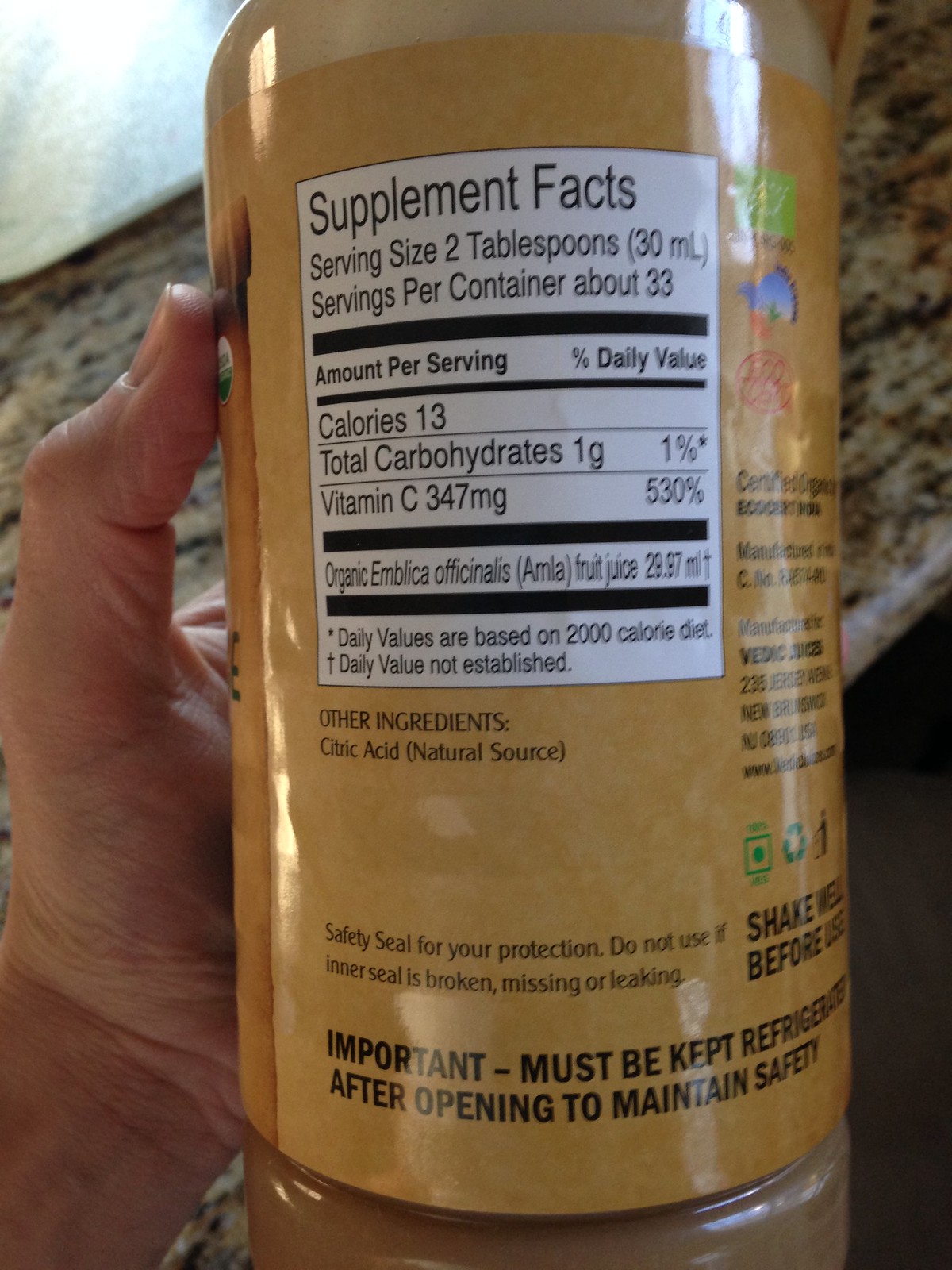A close-up color photograph taken indoors, featuring a hand holding a bottle with the focus on the back label. The label has a light brown background with a black pencil-outline section highlighting nutritional information. It indicates "Supplement Facts" with a serving size of two tablespoons (30 milliliters) and approximately 33 servings per container. The label lists "citric acid" under "Other Ingredients," noted to be from a natural source, and advises to "shake well before use." The bottle appears to contain a brown liquid, suggesting it might be a chocolate-based product. The hand holding the bottle is white-skinned, with the left thumb supporting the side. The background reveals a kitchen countertop with a distinctive brown and black granite pattern, hinting that the photo was taken in a home setting.